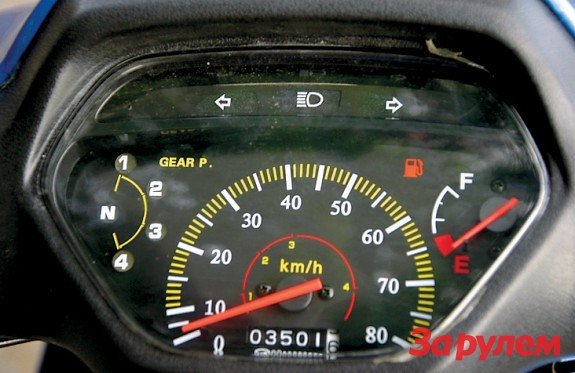The image captures a detailed view of a motorbike's speedometer, prominently displayed within a sleek black casing. The dial reads in kilometers per hour, with the needle resting just slightly above zero, indicating that the bike is either stationary or just beginning to move. At the top of the display, there are clear indicators for left and right signaling, as well as the high beam headlights.

To the right of the speedometer, a fuel gauge is visibly empty, accompanied by a warning light alerting the rider to the low fuel level. On the left side of the display, the gear indicator shows the positions for gears one through four and neutral. 

The odometer at the bottom of the speedometer reads 3,501 kilometers, suggesting the distance traveled by the bike. A small label in the corner reads "3A," and another possibly indicating either a different language or a company name remains partially obscured.

The surrounding elements and a glimpse of blue hint at the color of the bike itself, making this a comprehensive snapshot of the essential controls and status indicators crucial for safe and efficient riding.